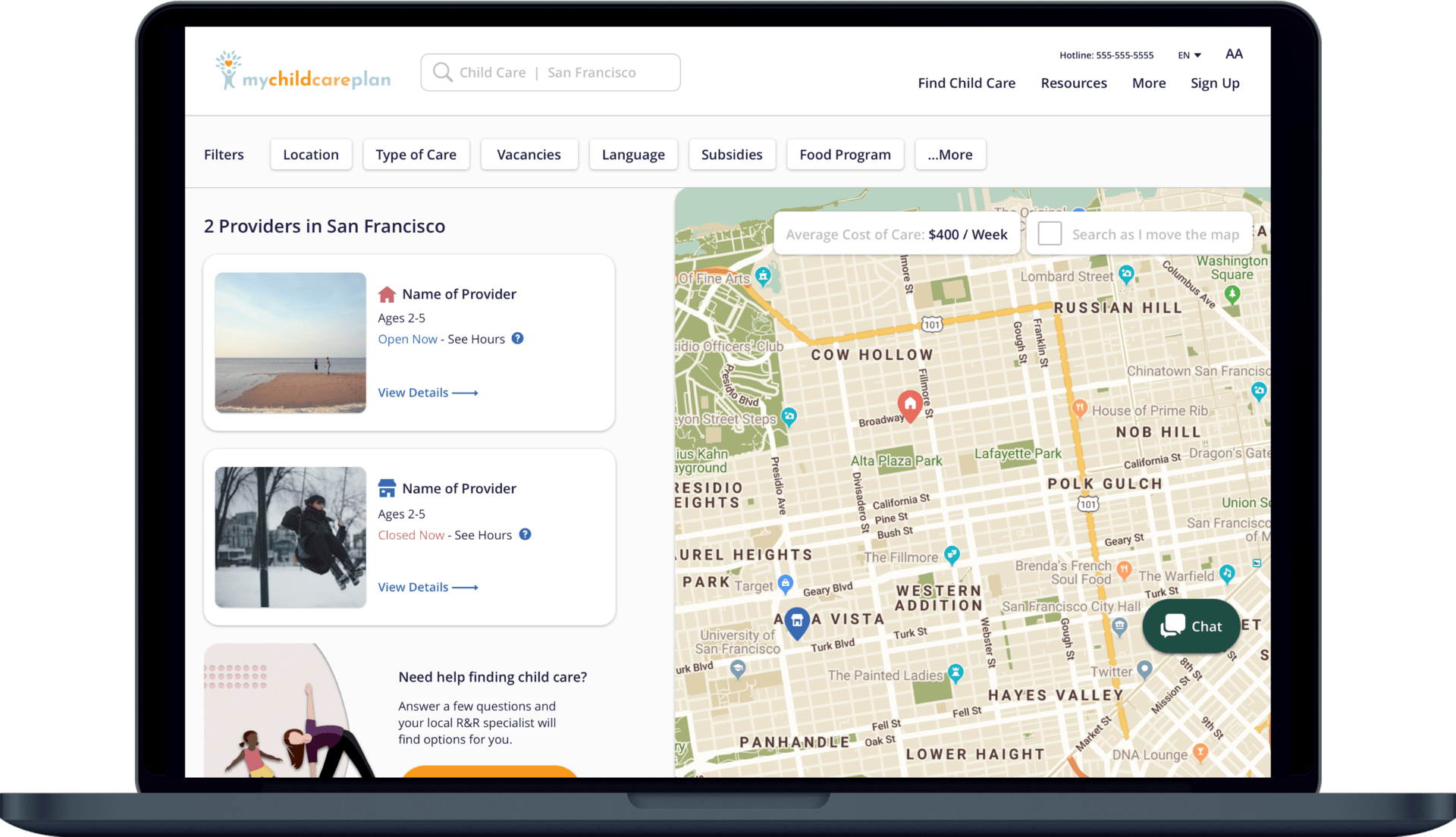On the laptop screen, the interface displays "My Childcare Plan" prominently at the top. Adjacent to the title is a logo depicting a child with a radiant heart or sun above them, symbolizing nurturing care. To the right of the logo is a search box labeled "Find Childcare Resources," accompanied by options to "Sign Up" and find "More."

Below the header, a navigation bar presents various filters for refining searches, including "Location," "Type of Care," "Vacancies," "Language," "Sub Cities," "Food Program," and more. Underneath the filters, a statement indicates there are two childcare providers available in San Francisco.

The page then displays search results in a box format. Each result includes the name of the provider, the age range they cater to, and their availability status, such as "Open Now." One search result features an image of a beach, while another showcases a child on a swing in the snow, bundled up in winter clothing. "View Details" links are provided in blue for more information on each provider.

Further down, the page offers assistance with a section headed "Need Help Finding Childcare," followed by some unreadable text and an orange button. To the left of this section is a clip art graphic of a woman stretching with a child, adding a playful element to the design.

On the right side of the screen, an interactive map highlights the locations of various childcare facilities, marked with pins. Above the map, search bars allow users to filter results by the weekly cost of childcare. A chat bubble in the bottom-right corner invites users to chat with support for additional help. The map itself occupies the majority of this section, providing a visual representation of the available childcare options.